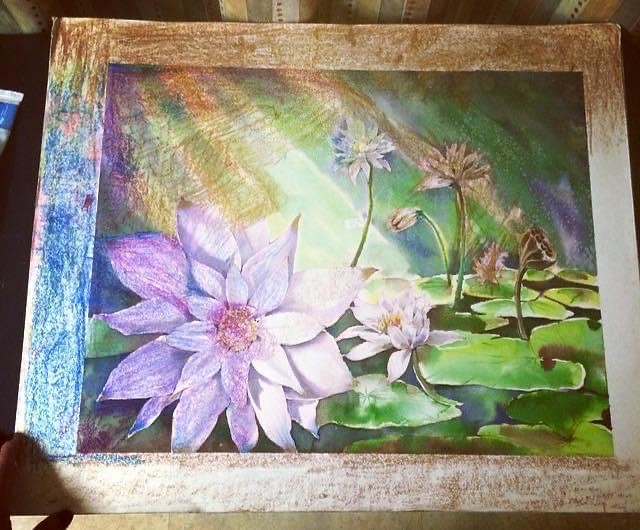This image captures a detailed close-up of a color drawing, showcasing various artistic techniques. The centerpiece of the drawing is a large purple lotus flower, depicted with intricate shading in light and darker purples. Surrounding its spindly center, the flower's petals are meticulously colored. In the background, additional flowers of smaller sizes in shades of purple and brown are visible, accompanied by green stems protruding from the depicted water. Green lily pads are scattered throughout, highlighted with white to emulate light reflections.

The drawing features a multi-colored penciled frame: the top part is scribbled brown, transitioning to white along the right side, the bottom is shaded with a mix of brown and white, and the left side features blue scribbles. A portion of a white hand, possibly part of the artist’s fingers, appears on the left side of the drawing, indicating they are interacting with the artwork, possibly touching it. The background within the frame shows a rough texture, suggesting the use of crayons, colored pencils, and possibly watercolors, as indicated by visible pencil or crayon strokes.

Additionally, there is part of a tube of paint lying on a brown table to the left, adding to the scene’s artistic context. The entire drawing is bordered by black, emphasizing its frame and separating it from the external environment. The combined elements make it look like a photo of a detailed, multi-media color drawing, illustrating both the flower and its natural pond habitat in one cohesive visual narrative.